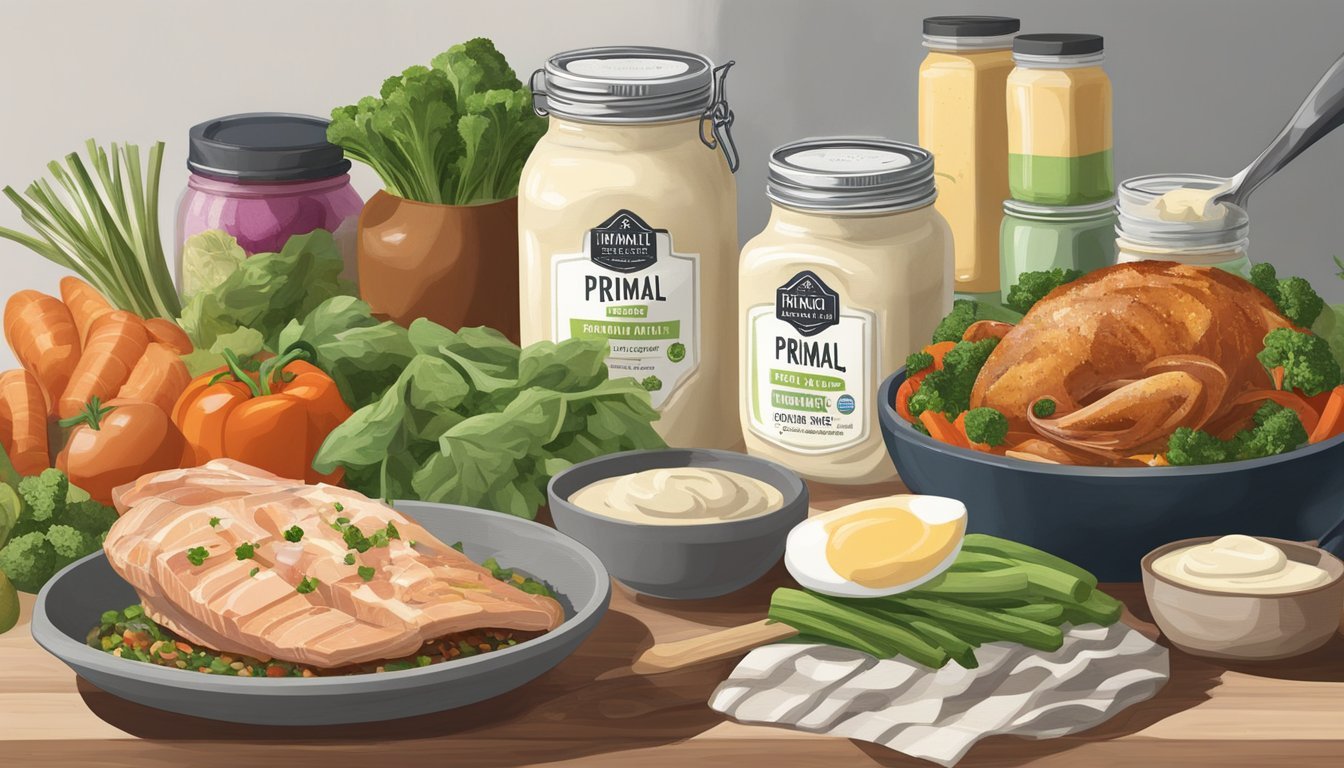This image appears to be a detailed and colorful illustration of a culinary spread set on a light brown wood table. In the bottom left corner, a gray plate holds a fillet of salmon or chicken breast, garnished with green parsley and accompanied by a colorful arrangement of vegetables, likely including couscous in shades of green, yellow, and orange. Behind this plate, an assortment of fresh vegetables such as peppers, tomatoes, lettuce, broccoli, carrots, and green onions is scattered across the table.

Prominently featured are two jarred containers labeled "Primal," one with a collapsed metal lid, and the other with a screw-on lid, hinting at them possibly being jarred mayonnaise. In front of these jars, two sauce cups containing different types of sauces are placed—one dark gray and the other light brown, blending with the table's color.

On the right, a browned roasted chicken, possibly a Cornish hen, is displayed in a grayish bowl, surrounded by bright green broccoli, carrots, and additional bunches of parsley. An egg cut in half is resting in front of the chicken, potentially on a bed of asparagus or other greens.

Also on the table are various containers and jars, including a tall yellow jar, a smaller two-toned jar with a yellow top and green bottom, and an open jar with a spoon sticking out of it. A brown jar with green lettuce-like leaves emerging from the top and another jar with a black lid, filled with a purple substance, contribute to the vibrant table setting.

Overall, the scene depicts a celebratory feast, showcasing the versatility of the displayed ingredients and the featured Primal-labeled jars.